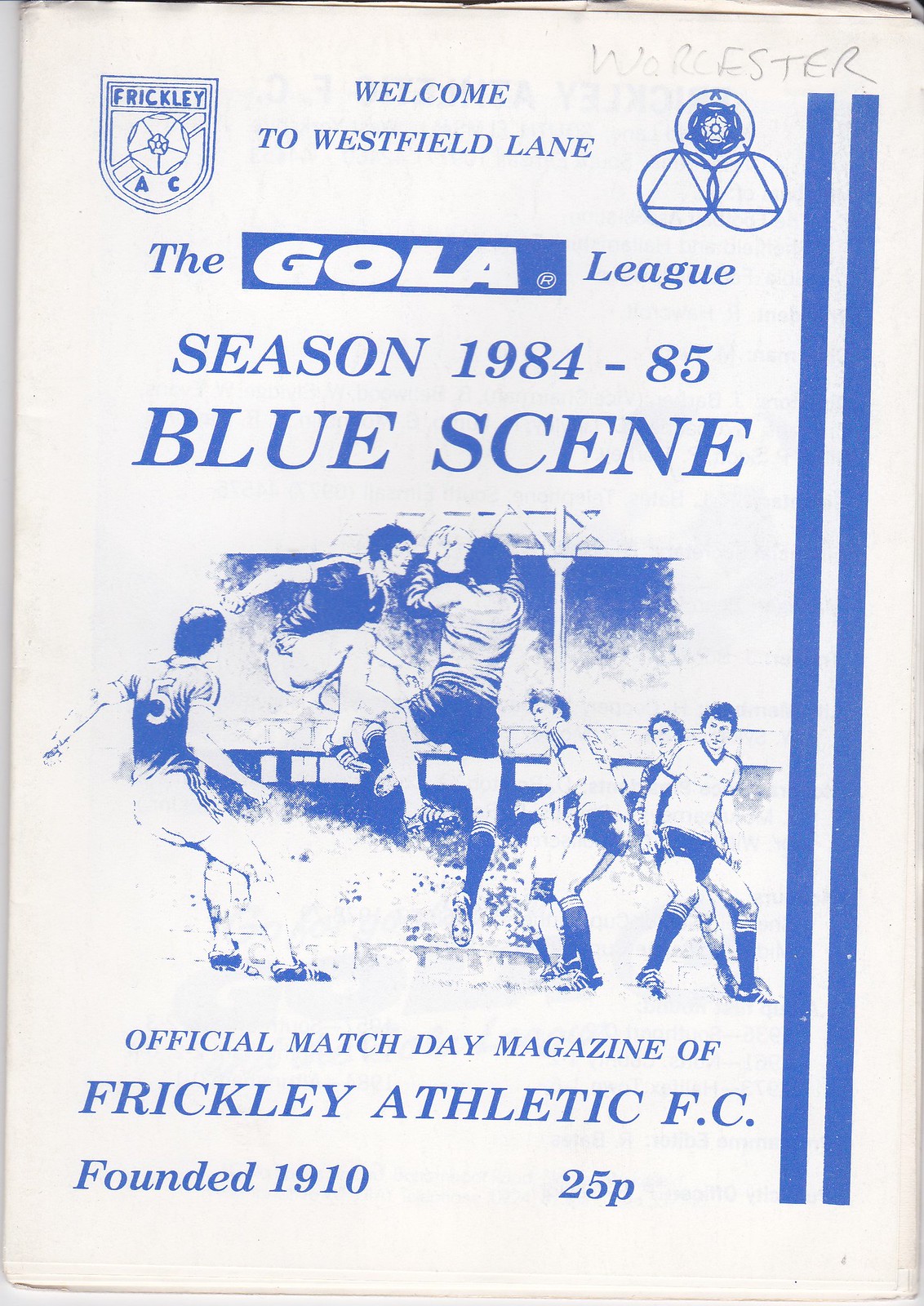The image is a vertically aligned rectangular picture of an aged booklet cover. It features a worn, white cover with two thick vertical blue stripes running down the right side. At the top center, the booklet's title reads in blue, all-caps letters: "WELCOME TO WESTFIELD LANE." Below, it continues with "THE GOLA LEAGUE," "SEASON 1984-85," and "BLUE SCENE." The middle portion of the cover displays a blue-and-white illustration of several soccer players. Two players are airborne with one player holding a soccer ball, while four others are grounded. The background hints at a field setting. Beneath the illustration, it states, "OFFICIAL MATCHDAY MAGAZINE OF FRICKLEY ATHLETIC FC." Additional text in blue at the lower left corner reads, "FOUNDED 1910," and on the lower right, "25P." The overall design evokes a nostalgic feel, enhanced by the brown, uneven edges of the paper.